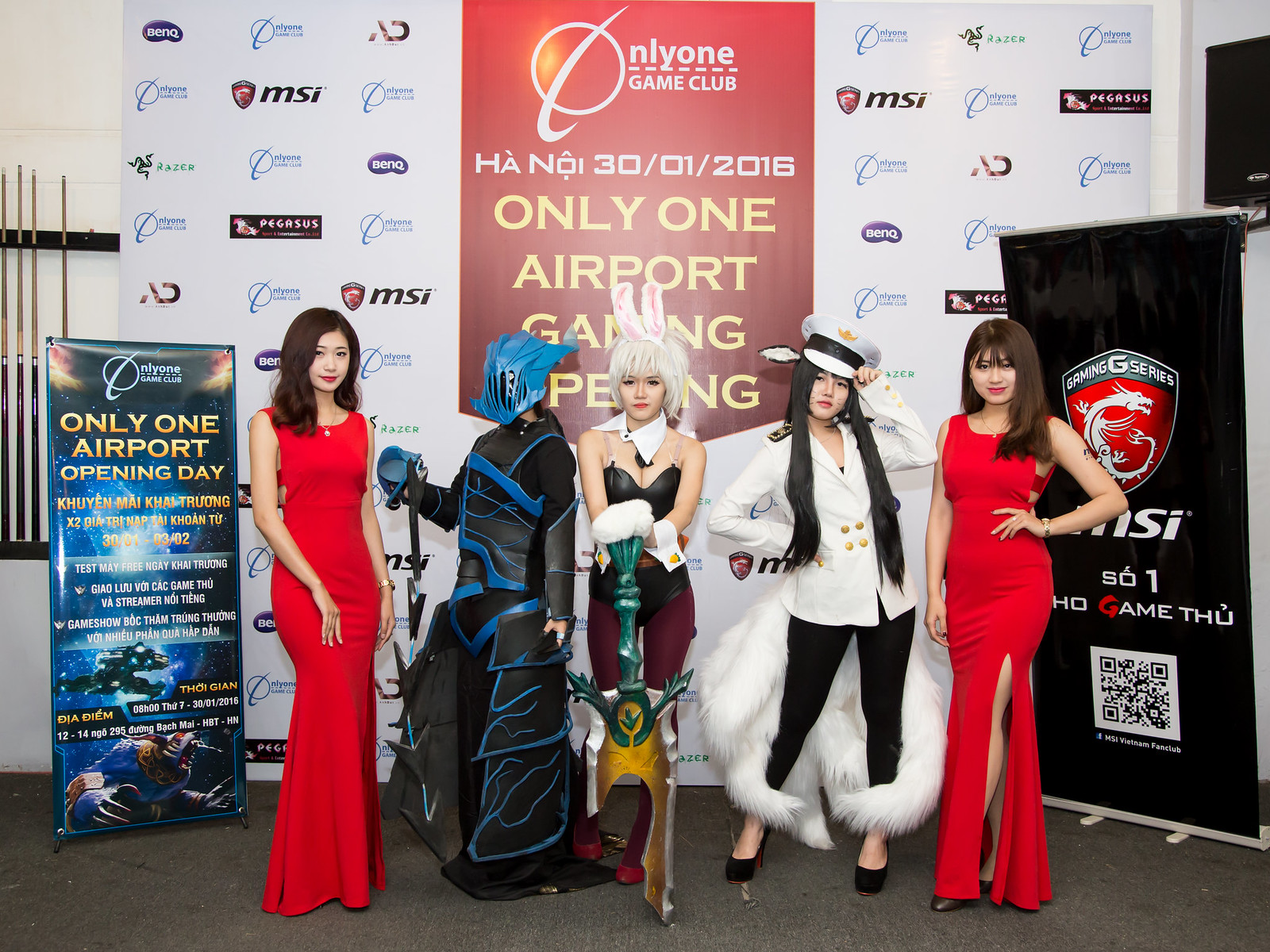In this bustling image from a cosplay event dated January 31, 2016, in Hanoi, five women stand prominently in front of a large white banner adorned with various sponsor logos such as MSI, Pegasus, BenQ, Razer, and AD. The banner bears an orange center logo with "Only One Game Club" and details of "Only One Airport Gaming Opening," flanked by smaller vertical banners showcasing galactic and gaming themes.

From left to right, the first woman wears a sleeveless red gown, a wristwatch, and has short shoulder-length hair, looking directly at the camera. Beside her is a character in a blue and black armor-like cosplay, with a fully covered blue helmet and wielding a weapon. Central to the group is a woman dressed as a bunny-themed character with white hair, bunny ears, a black corset with purple accents, and white gloves, holding a colorful enameled sword. To her right stands a woman in a naval-inspired outfit featuring a white captain's hat, jacket with epaulets, black pants, and heels, with her hand on her waist and a fur tail draping from behind. Finally, the woman on the far right mirrors the first with a shoulder-length hairstyle, red slip gown, brown high heels, and a wristwatch, completing the ensemble with a tattoo on her arm. The scene is framed by a vertical gaming-themed banner to the left and a black poster with a red dragon logo to the right.